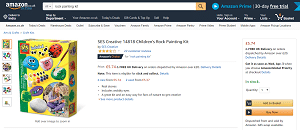The image is a somewhat blurry screenshot of the Amazon homepage. The top part of the screen is in a navy blue color, featuring the iconic white "Amazon" logo on the left-hand side. Adjacent to the logo is the word "Prime" in blue, accompanied by the orange Amazon arrow pointing right.

Below the header, there's a search box predominantly white in color, with the right-hand side transitioning to orange. On this orange part, a black magnifying glass icon is visible, signifying the search function. The text within the search box is black but illegible due to the blur.

To the right of the search box, there's a white-and-blue circular icon. This circle displays something in white with the word "Prime" in blue and the text "30-day" following it, though the rest of the text is unclear.

The bulk of the image seems to showcase a product - a colorful box predominantly yellow with a green section on the left side. The product appears to be a painting kit for rocks. Though the text on the product is unreadable due to the blur, the picture shows painted rocks, suggesting that the kit includes both paint and brushes, probably with rocks for decoration. Visible painted designs include a ladybug, a pig, a blue face with a mask, and a green shamrock.